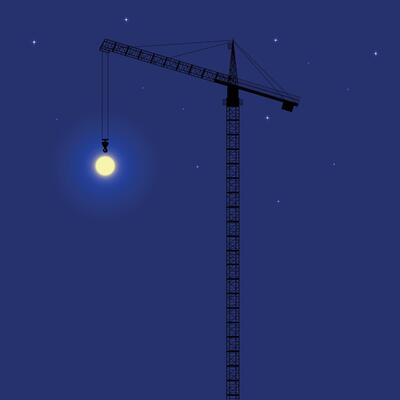In this nighttime outdoor image, a towering construction crane, characterized by its skeletal structure of steel bars welded into rectangular frames, dominates the view against a deep indigo sky. The crane, standing tall and tapering to a point, intersects the picturesque expanse filled with sprinkled clusters of white star-like dots. At the crane’s apex, long cables extend, connecting the top to both the hefty counterweight and the operational front end. From this operational end, a black tether dangles, terminating in a piece reminiscent of an upside-down chess piece. Just below this tether, the luminous, yellowish moon with a hazy white halo, adds a celestial touch to the scene, positioned slightly left of center. The crisp, cloudless sky intensifies the overall blue hue, creating a stark contrast with the crane’s dark silhouette, crafting an atmospheric, construction-themed nightscape.